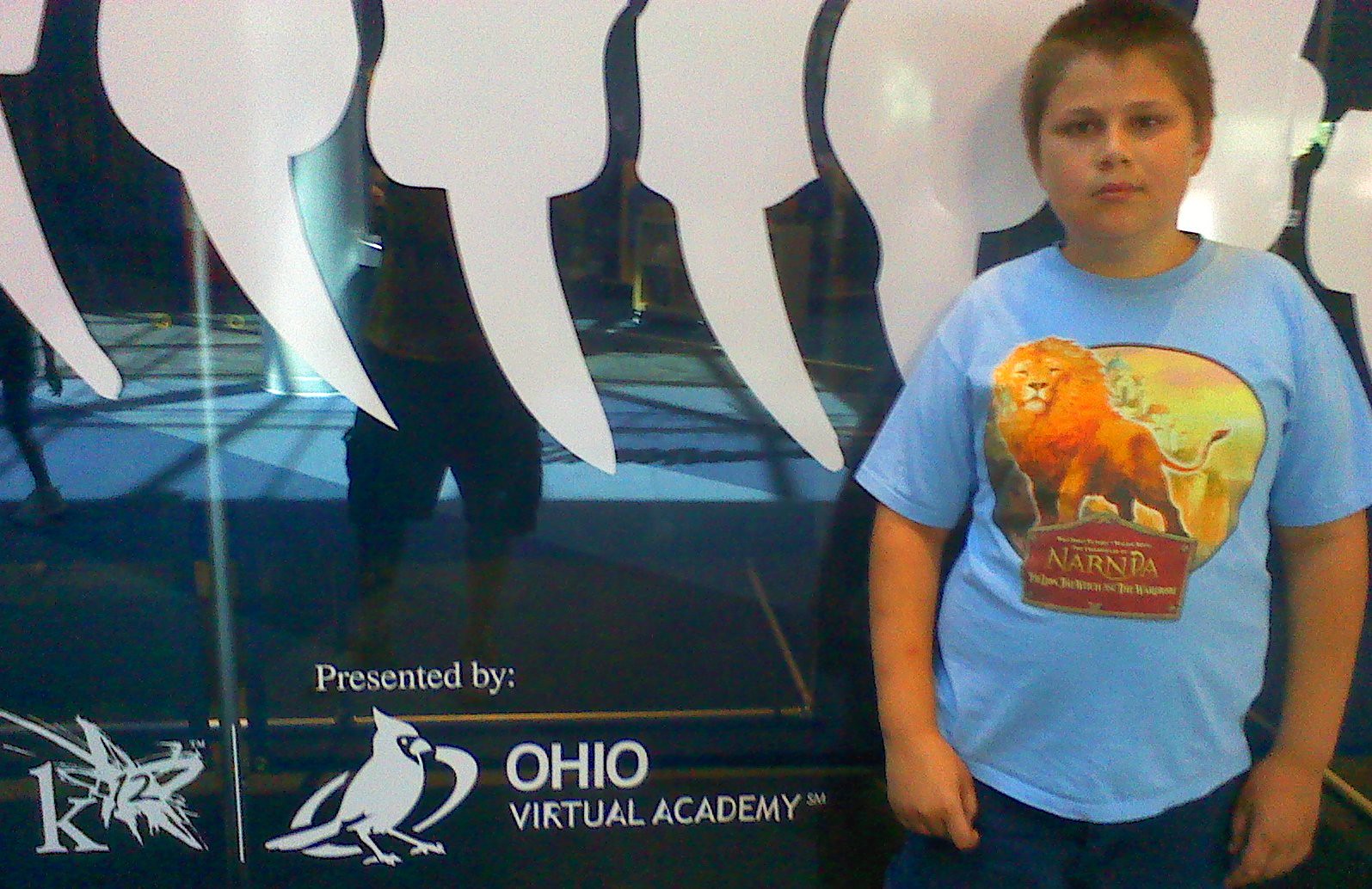In this image, a young Caucasian boy with short brown hair stands in front of a metallic, reflective display at what appears to be a library or museum. Positioned in the right third of the horizontal rectangular frame, he is wearing a blue t-shirt featuring a prominent lion image from the Chronicles of Narnia with the word "Narnia" beneath it. The boy wears dark blue shorts and has his arms resting at his sides, looking straight at the camera with a neutral expression.

The background display behind him is black and shiny, adorned at the top with a series of white, comma-like shapes that extend horizontally. At the bottom of the display, in white text, it reads, "Presented by Ohio Virtual Academy," accompanied by a logo of a cardinal encircled. Additionally, the text "K-12" is visible at the bottom left of the display. The reflection of the photographer, possibly an adult male, can be seen in the reflective surface.